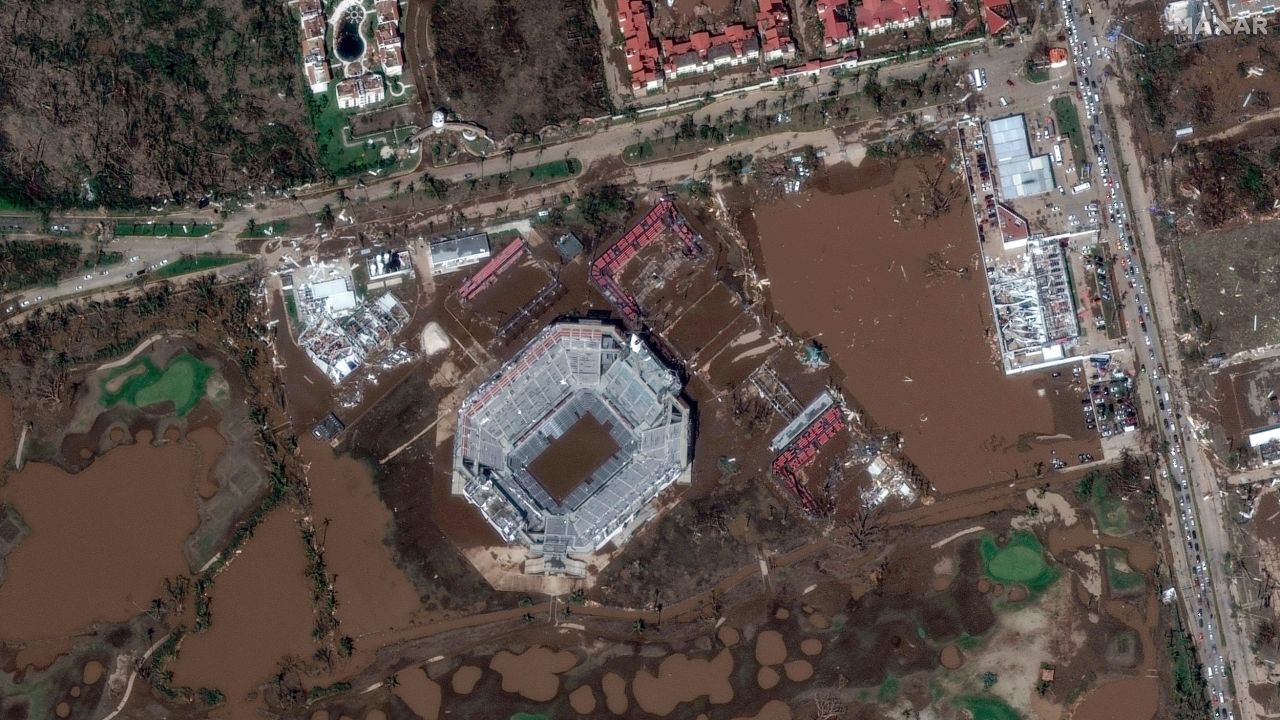This aerial photograph showcases a football stadium prominently situated amidst a surrounding landscape characterized by expanses of brown dirt that vary in shade. The stadium features a rectangular field with a distinct brown hue at its base, encircled by gray bleachers forming a loose hexagonal shape. Notably, the stadium appears empty, suggesting no event is taking place at the time of the capture.

Encircling the stadium are various roadways filled with numerous cars, emphasizing the connectivity of the venue with its surroundings, and hinting at bustling activity despite the apparent stadium inactivity. The roads are predominantly positioned to the right of the frame, interspersed with assorted buildings.

Further beyond the immediate vicinity of the stadium, the image captures both residential and urban structures. The rooftops of these houses are visibly red, contrasting against the darker brown dirt that encapsulates their neighborhood. Overall, despite the presence of infrastructure, the overall ambience of the photograph is dominated by the earthy, brown tones of the surrounding landscape, which add an intriguing contrast to the organized structure of the stadium and adjacent roadways.